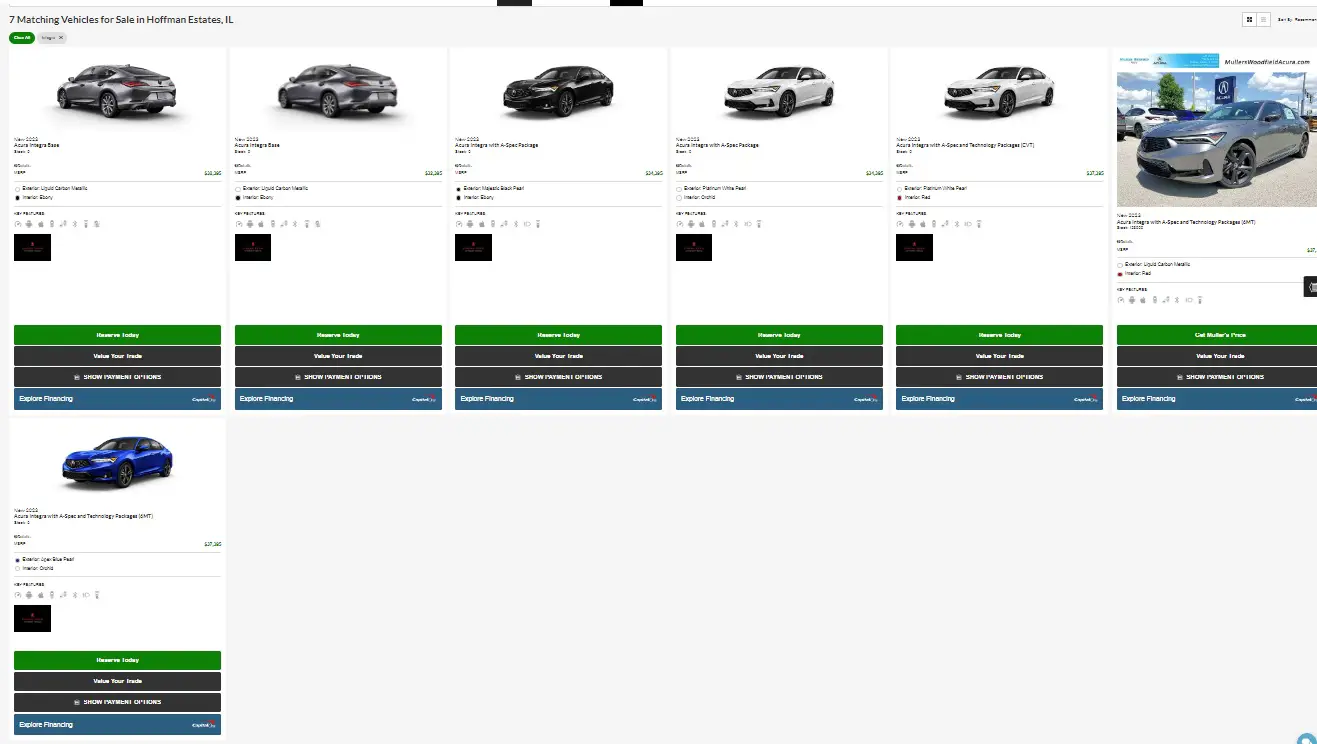At Hoppin' Estates in Green Oval, there are 7 matching vehicles for sale. The description highlights the following details:

1. The first vehicle appears in a black and silver color scheme.
2. The second vehicle is gray.
3. The third vehicle is black, and the view showcases its front.
4. The fourth vehicle is an Acura Integra equipped with the A-Spec package.
5. The fifth vehicle is an Acura Integra featuring both A-Spec and Technology Packages.
6. The sixth vehicle is yet another Acura Integra with both A-Spec and Technology Packages.
7. The seventh vehicle is a blue Acura Integra with A-Spec and Technology Packages. It boasts an exterior in Blue Pearl and an interior in Orchid.

Notably, some vehicles have alternate interior color options including red and ebony, and exteriors in Platinum Pearl, Black-Brown, and Liquid Carbon Metallic.

Additionally, Green Oval Estates, the sales venue, is currently reserved by HRH and financing options will be available through Jens Explore Financing. This message is prominently repeated.